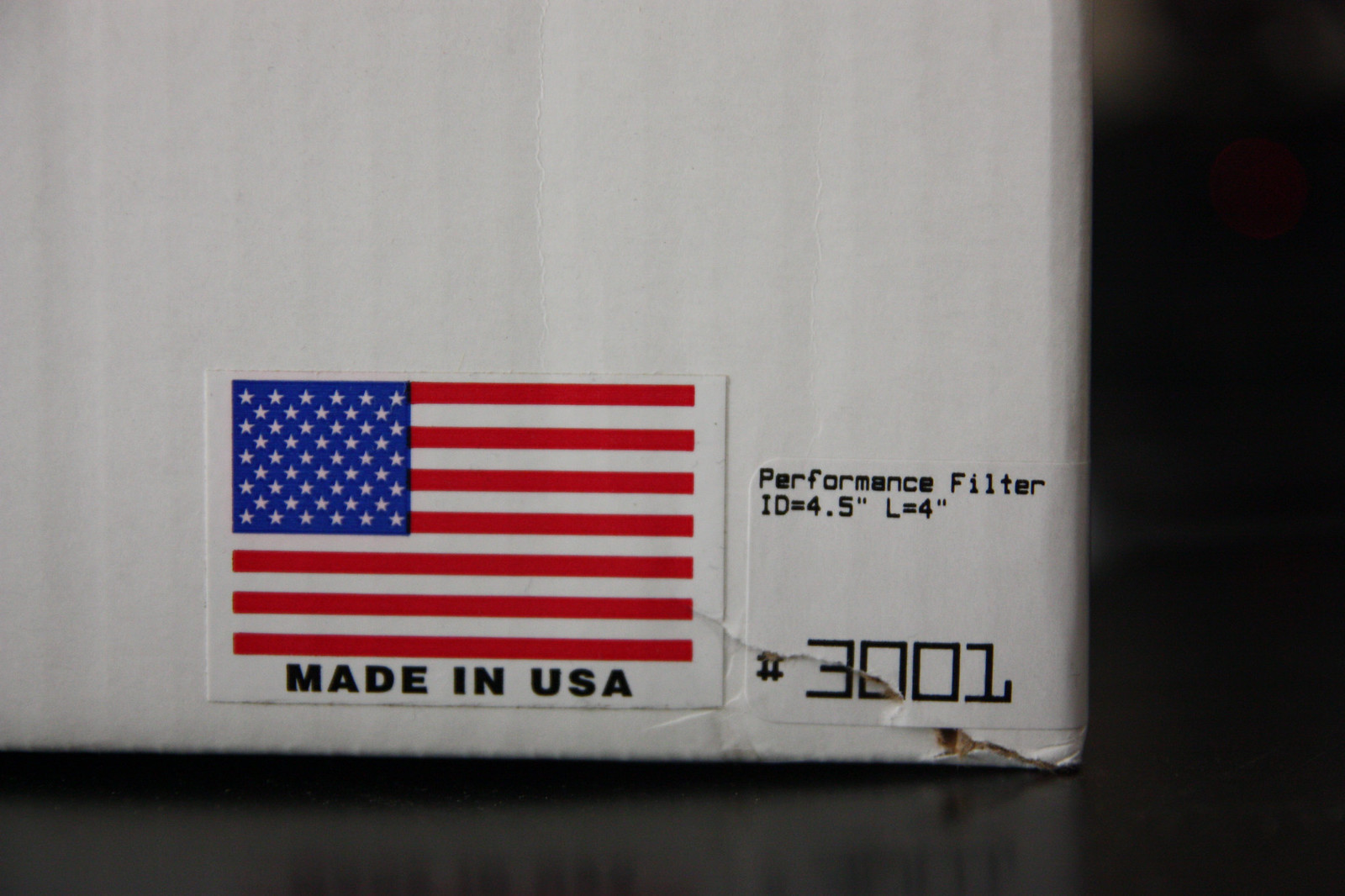In this image, a partial view of a white box is displayed, with only the bottom corner visible. The remainder of the box is not shown. The backdrop is a blurred black, adding no additional context. On the left side of the box, there is a sticker of an American flag, featuring red, white, and blue colors, with the words "Made in USA" printed in bold black beneath it. Adjacent to this, on the right side, is another sticker. This one reads "Performance Filter" at the top and "ID = 4.0" below. The image's focus on these details suggests the box is likely related to a specific product, potentially an automotive or mechanical component given the nature of the stickers.